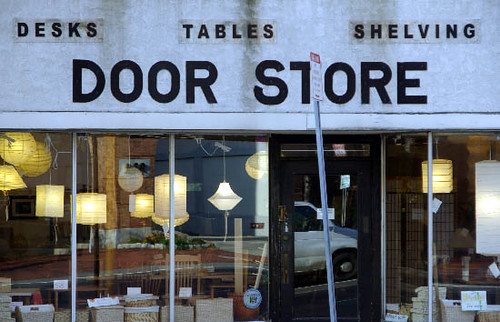The image captures a horizontally rectangular storefront, viewed from a slightly elevated angle just above ground level. The lower section of the frame predominantly features expansive windows, segmented by thin, vertical silver frames. A doorway, positioned centrally and framed in a deep dark brown or possibly black color, divides these window panes. Ascending to the upper portion of the frame, the exterior wall of the store presents a clean, light gray surface. Prominent signage adorns this facade, with smaller text along the top spelling out "Desks, Tables, Shelving." Below this, in substantially larger and more commanding letters, the store's name, "Door Store," is prominently displayed.